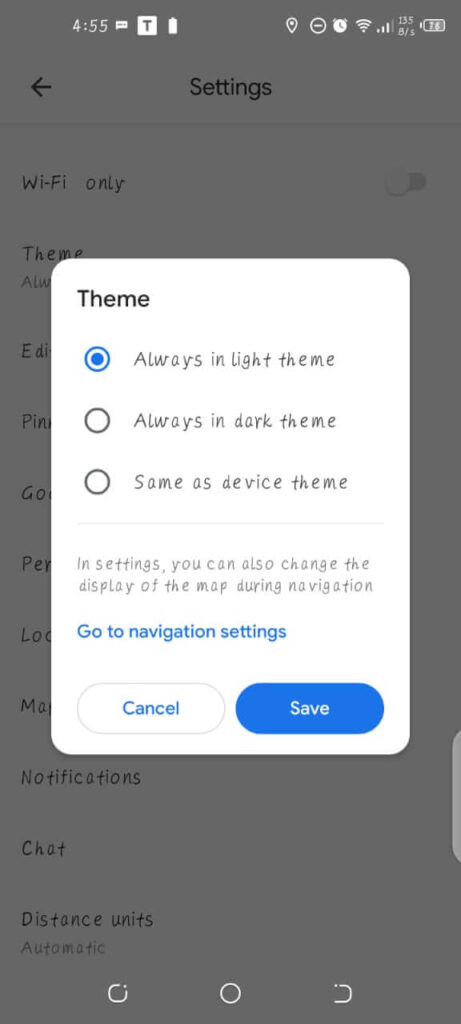A settings interface is displayed on a smartphone with a medium gray background. 

At the top of the screen, the status bar shows various icons. On the left, it reads "4:55" in white text, followed by a white square with a gray "T" inside it. Next to it, an unclear icon that might be a trash can or discard icon is visible. On the right side, standard icons are displayed: location, ringer or alarm, Wi-Fi, signal strength, and battery charge, which appears to be around 70%.

Below the status bar, in black text against the grayed-out background, it reads “Settings” with a left arrow to return to the previous screen. The visible options below are "Wi-Fi only" and "Theme." Additional options are partially obscured, labeled "ED..." and "PIN..." followed by "GO...".

The central focus is a white overlay labeled "Theme" in black text. This overlay contains three radio buttons, each options for theme settings:
1. "Always in light theme" – selected and highlighted with a blue circle.
2. "Always in dark theme" – unselected.
3. "Same as device theme" – unselected.

A thin horizontal line separates these options from additional text that reads, “In settings, you can also change the display of the map during navigation." Below, in bold blue letters, it says “Go to navigation settings.”

At the bottom of the overlay are two clickable options. The left is a gray-outlined oblong button with “Cancel” in blue letters, and the right is a solid blue oblong button with “Save” in white letters.